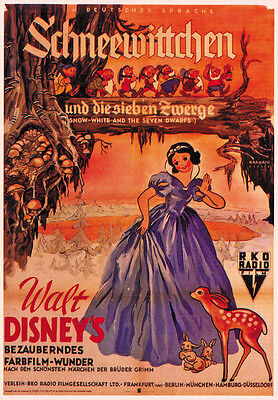This is a vintage German advertisement poster for Walt Disney's "Snow White and the Seven Dwarfs," titled "Schneewittchen und Die Sieben Zwerge." The film's title is prominently displayed in German, with "Walt Disney's" in red lettering above it. The central figure is Snow White, depicted in a purplish-blue dress, standing next to a small deer and several rabbits. The background is dominated by a fantastical tree with mushrooms and smaller trees, creating a lush forest scene. The seven dwarfs are happily marching across a wooden bridge made from another tree, illustrating their whimsical journey. The color palette of the poster is primarily shades of reds and browns, enhancing its vintage appeal. Additional fine print mentions Berlin and Frankfurt, indicating the regional focus of the advertisement.